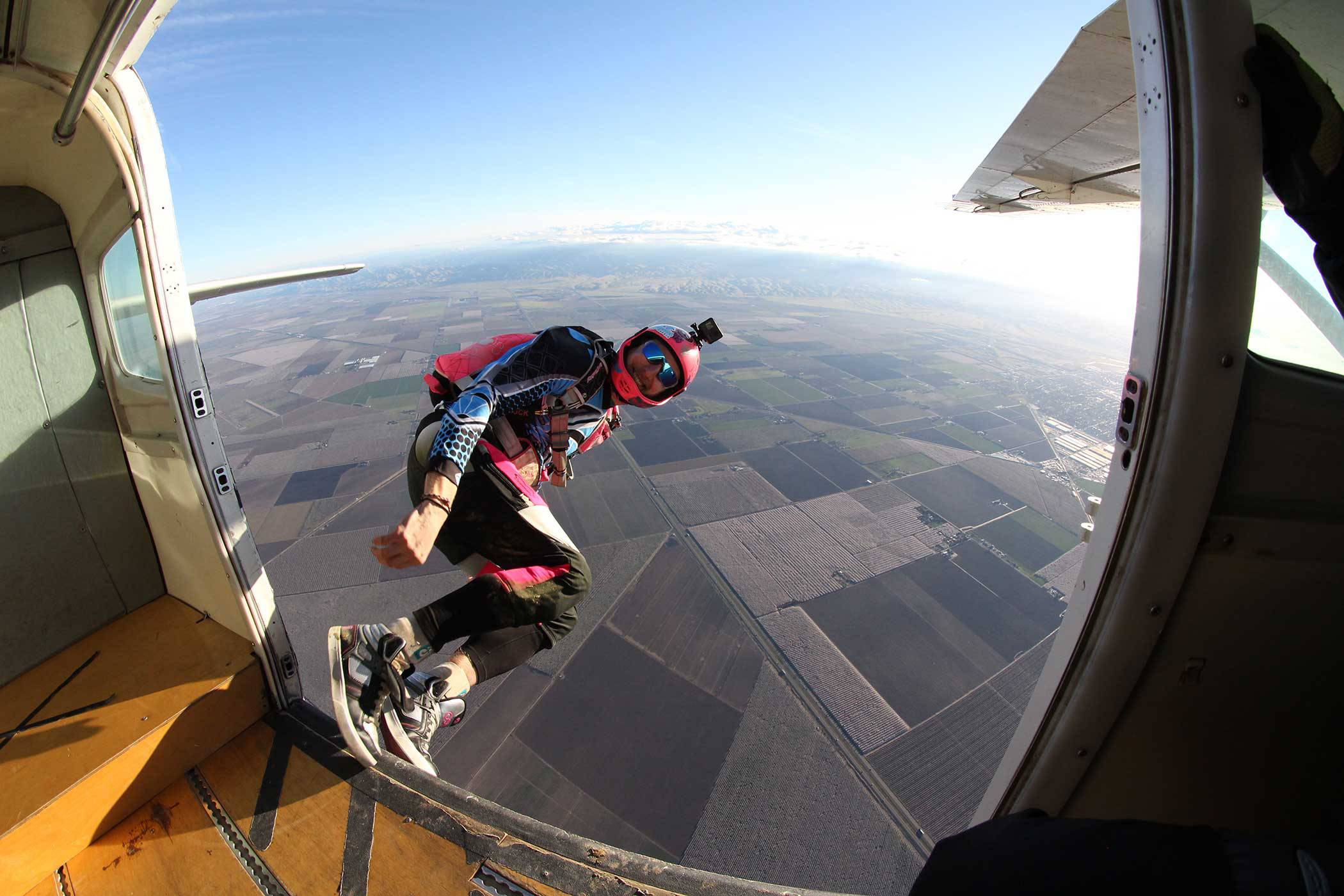The image captures a thrilling moment from inside a moving airplane on a bright, clear day with a blue sky. A person fully geared up is mid-jump out of the open cabin door of the plane. The individual, adorned in a black and blue compression outfit with long sleeves and black compression pants featuring a red stripe, is stepping off the yellow and black-taped floor of the aircraft. The jumper is equipped with a red helmet, mounted with a GoPro camera, and is wearing distinct white and black sneakers. He carries a hot pink parachute on his back, which matches the red accents on his helmet and outfit. His face, partially obscured by blue sunglasses, shows him smiling back towards someone inside the plane. The airplane's interior is also visible, featuring a wooden floor with no seats, and the wing of the aircraft edges into the top right corner of the frame. Below, a patchwork of brown and green farmland stretches out, interspersed with roads and varying tracts of land, all under a vast, open sky devoid of clouds.